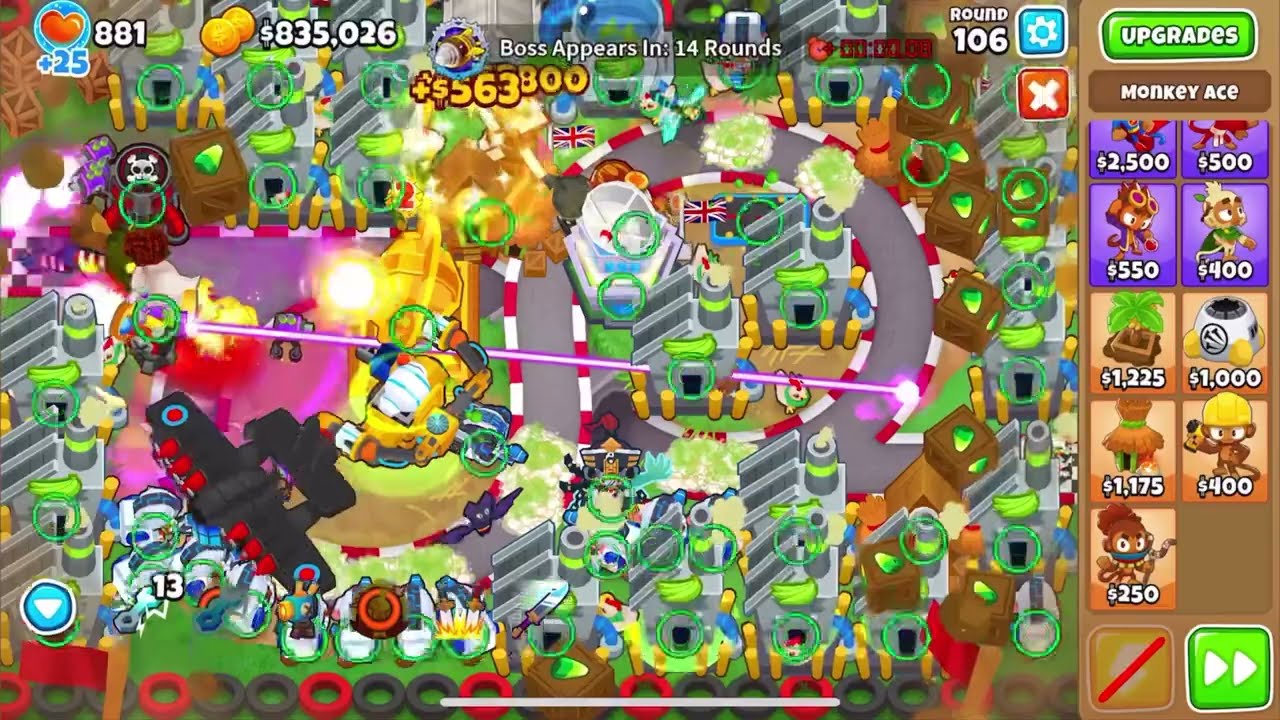The image is a vibrant, colorful screenshot of a tower defense game. Dominating the left and center is a yellow car and a black jet with elongated rectangular wings, firing lasers across the frame. Red dots appear in front of the wings, and on the top left, a heart icon shows "+25", alongside the current health displayed as "881". 

The right side of the image features a prominent "Upgrades" menu. This menu includes various purchasable items such as "Monkey Ace" within a green rectangle with white outlined text. Several upgrade options are listed below, each with distinct prices: a $2,500 option, followed by $500, $550, $400, $1,225 with a palm tree icon, $1,000 with a white circle, and $1,175. There's also a monkey character with a yellow hard hat priced at $400, and a girl monkey with a ponytail for $250. The menu's bottom section shows a red pen icon and a green button with rounded corners, containing two right-pointed triangles.

Additionally, in the bottom right corner, there's a detailed image of a black bomber plane flying over a track that looks like a road surrounded by buildings, underlining the game's strategic layout. An informational section indicates the current cash at $835,026, with text announcing "Boss appears in 14 rounds".